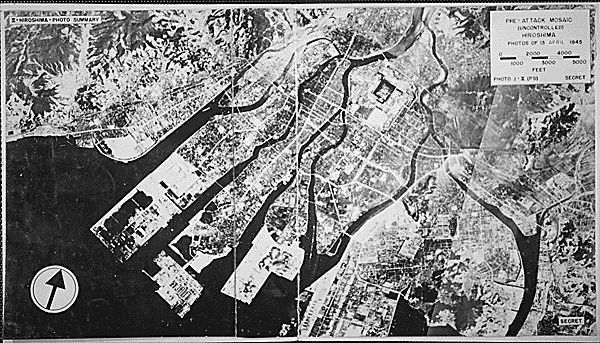We are looking at a black and white aerial photograph of Hiroshima taken in April 1945. The map is labeled "Hiroshima Photo Survey" and it has detailed annotations including "pre-attack mosaic," "uncontrolled," and "secret" in the bottom right corner. The image captures the city's layout, showing ports, rivers, roadways, and other land features from a very high vantage point, possibly from an airplane or satellite. An arrow within a circle points towards the land, indicating significant focus or reference. This photograph, marked "Photo 1-2," serves as a stark reminder of Hiroshima before the devastating attack that followed months later.